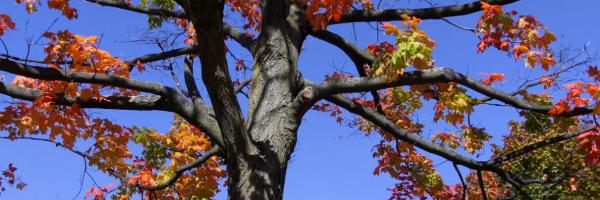This long, rectangular image, reminiscent of a bookmark, features a striking autumn scene viewed from the base of a tree looking upwards. The tree, potentially an oak or maple, displays a rough, predominantly brown bark highlighted by white reflections, giving it a slightly shiny appearance. The focus is on the tree's branches, which extend outward and are adorned with a variety of fall foliage—vibrant oranges, deep reds, pale yellows, and some remaining green leaves. These leaves create a picturesque contrast against a clear, cloudless, blue sky. Some branches appear to have been trimmed, adding a sense of past maintenance to the tree. In the background, the green foliage of a pine tree is faintly visible, adding depth and contrast to the scene. This image beautifully captures the essence of an autumn day.